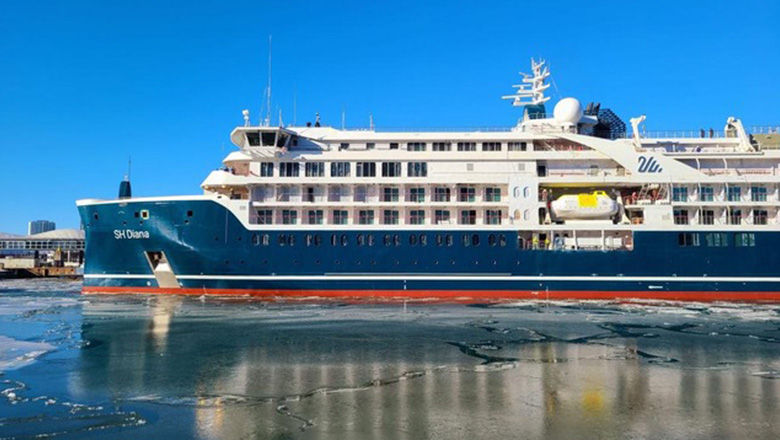The photograph captures a magnificent cruise ship named "S.H. Diana" docked at port. The vessel is primarily white with navy blue accents and features a distinctive red and white stripe along its bottom edge. The ship appears grand with multiple stories adorned with windows, sliding glass doors, and private balconies resembling cabanas. The sky is a brilliant, cloudless blue, reflecting the bright, sunny day. The foreground reveals crystal-clear water and a sandy shoreline, contrasting with the ship's vivid colors. A large building with numerous windows stands behind the dock. The ship is equipped with large antennas reaching skyward and there's a noticeable yellow square beneath the lifeboats on its side. Sparse activity is visible, with possibly one crew member near the lifeboats and two distant figures on the top deck. The serene and inviting atmosphere suggests the ship is either moored or approaching the port with its name, "S.H. Diana," prominently displayed on the bow.